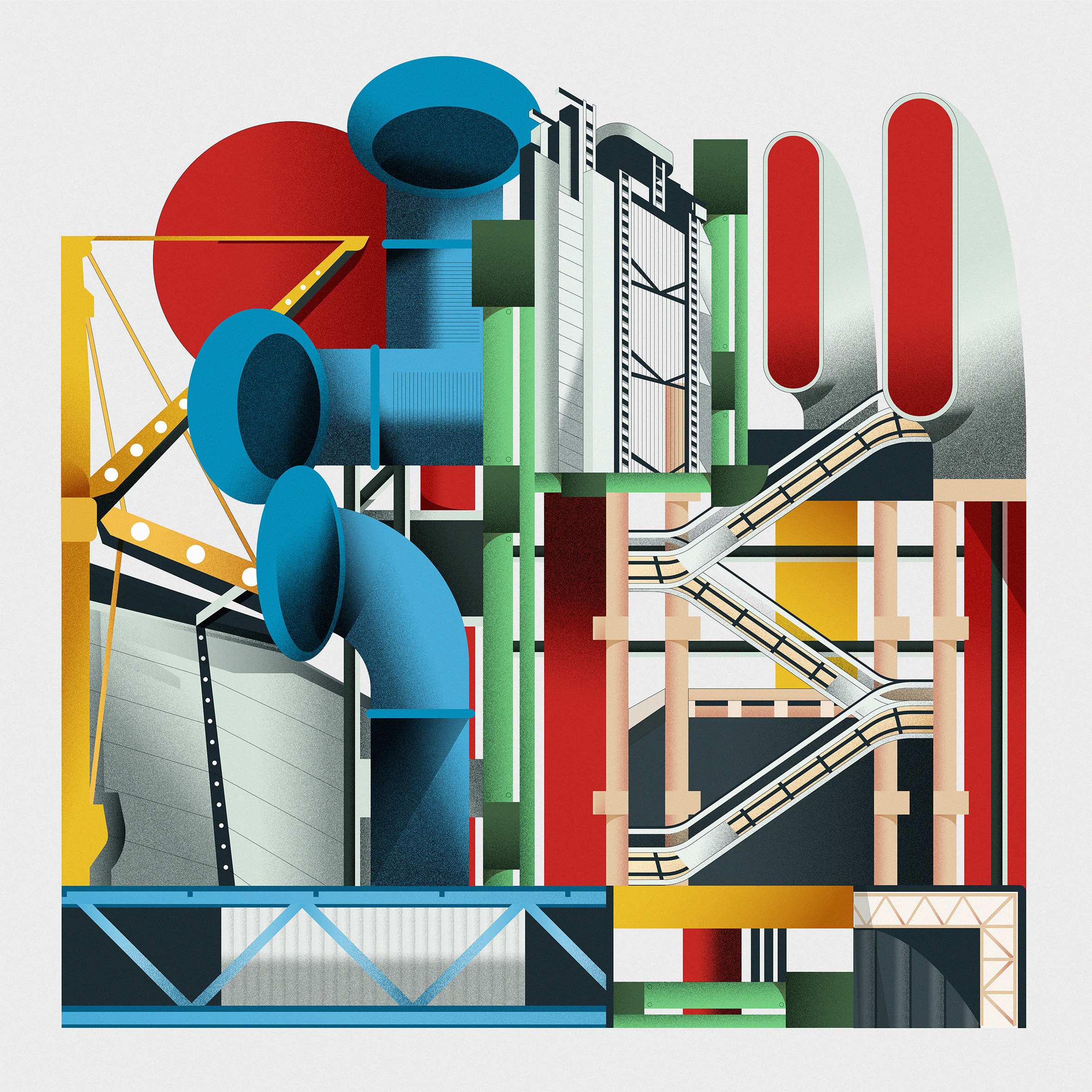The image is a vibrant and intricate Art Deco-inspired drawing with a light gray background, divided into four distinct sections. Layers of colors and shapes create a collage-like composition, showcasing a medley of industrial and architectural elements. Bright blues, dark blues, deep yellows, rich reds, and greens are prominently featured throughout, enhancing the complexity of the artwork. 

In the bottom right corner, vivid hues of yellow, red, and green form what appears to be a stylized shopping center, complete with escalators ascending to three levels, leading to the top right corner. There, gray chimney stacks with textured noise and bright red openings stand next to a pencil-like skyscraper in dark blues and grays. 

The bottom left corner displays a stylized pale blue steel girder, from which blue textured pipes and tubes rise. Tall green rectangular shapes and a yellow construction crane-like structure add to the industrial motif. A bright red circle, reminiscent of a sun, dominates the background in the top left corner, overseeing the entire scene. The artwork combines round and straight lines, with layered elements that invoke a feeling of mechanical assembly, leaving much to the viewer's interpretation.